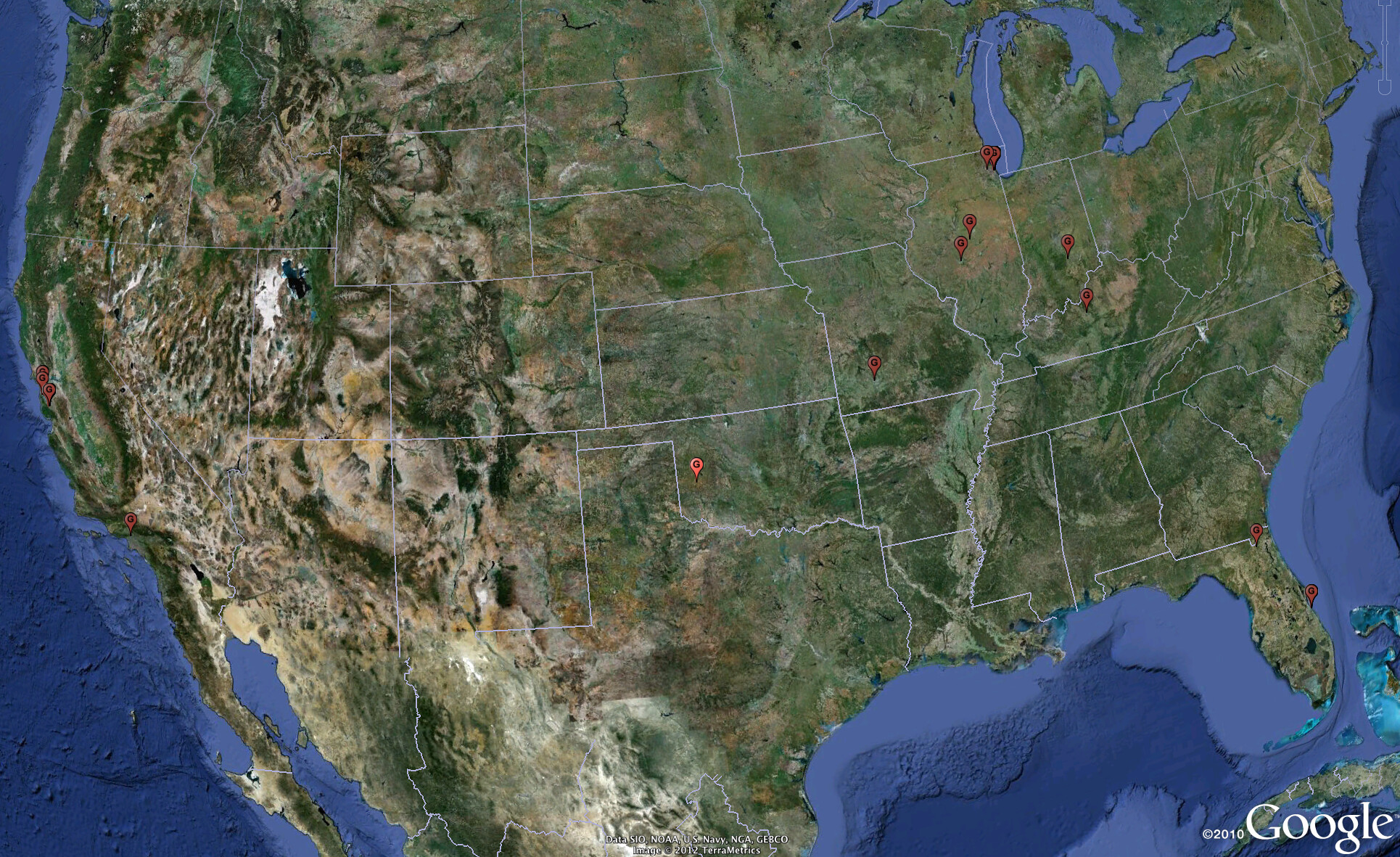This satellite image from Google Maps presents a detailed view of the United States. The map is accentuated with white lines that clearly delineate the borders of each state. Several pin drops highlight specific locations: one in Oklahoma, five clustered in the top left region around Ohio, Kentucky, Indiana, and Illinois, and two in Florida. The map is slightly angled towards the right, providing a dynamic perspective of the country. In the bottom left corner, the image is marked with "Copyright 2010 Google," indicating its source and year of creation.